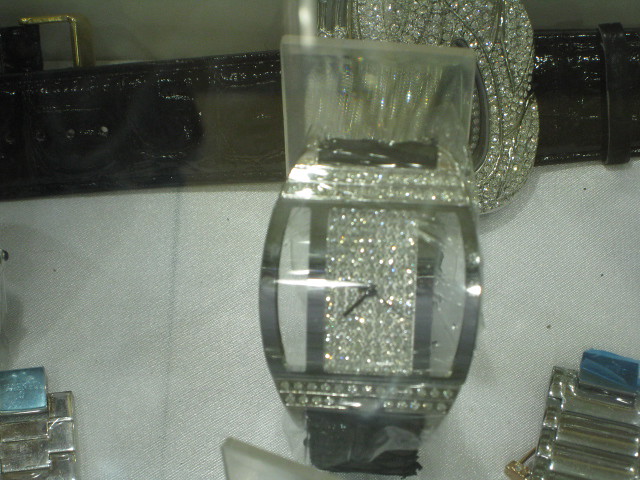The photograph captures an intricate, rectangular watch with an opulent design. The watch face, devoid of numbers, features three black hands set against clear glass and is bordered by a lavish arrangement of diamonds. The glass face is notably rectangular with curved edges and further bordered by black trim, complemented by additional diamonds lining both the top and bottom. The surrounding watch structure appears to be crafted from silver or platinum, enhancing its luxurious appeal. The watch rests on a white surface, partly overlaid by a black leather belt and accompanied by another piece of diamond-encrusted jewelry, which has a floral motif with a central black oval. Reflections from the silver watch bands are visible on both sides, contributing to the overall gleam of the scene.